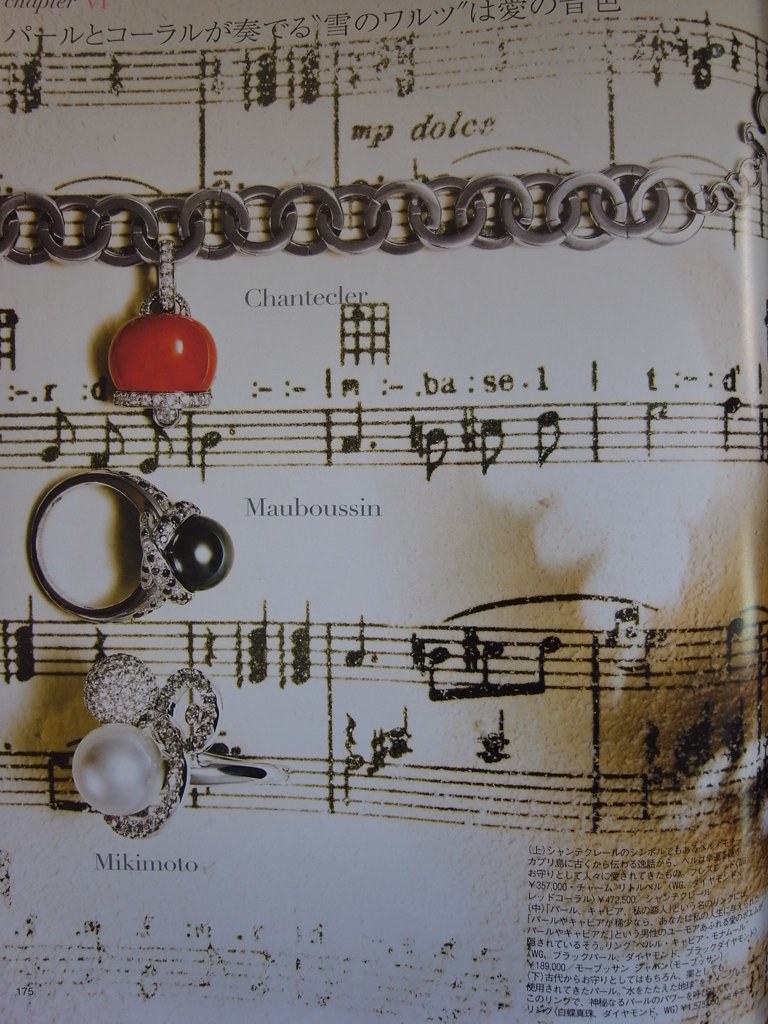In this photograph, the backdrop is a sheet of aged music paper, possibly from a magazine, with a glossy, curled edge on the right side. The sheet displays black musical notations on a white and slightly browned background. Draped across the second row of notes, there is a silver metallic chain, resembling a bracelet, adorned with a red charm encircled by diamonds. Just below this chain, lies a ring featuring a black stone. Farther down, there's an intricate piece of jewelry, which appears to be an earring with a central pearl surrounded by diamonds, and beside it, another decorative piece with three circular elements arranged to resemble the iconic shape of Mickey Mouse's head, featuring a large pearl in the central ring.